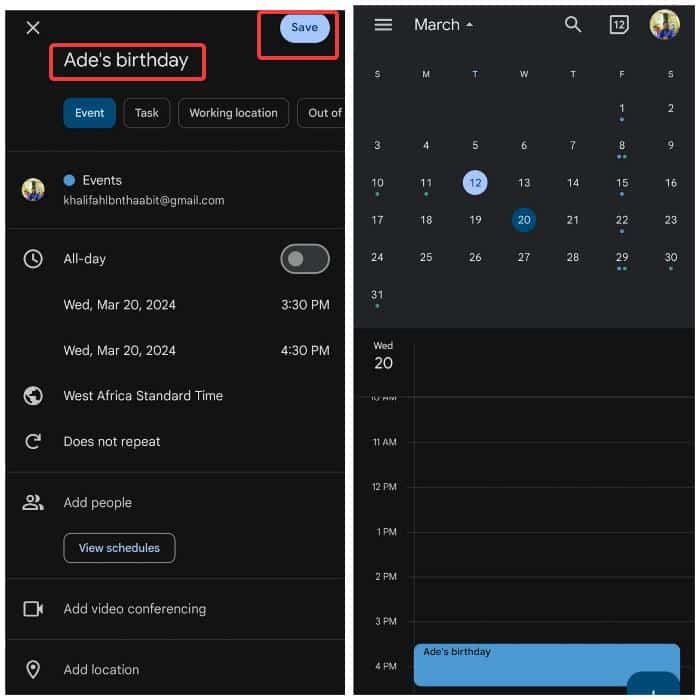Two adjacent mobile phone screenshots detail a calendar and events page.

**Left Screenshot:** 
- **Background:** Dark-themed with black backgrounds and white text.
- **Header:** At the top left is an 'X' to close. The top right features a saving button in a light blue or purple shade with black text, outlined by a somewhat uneven red rectangle.
- **Highlighted Sections:** The event label "AIDS Birthday" is surrounded by a red rectangle.
- **Navigation:** Below the header, a series of navigation buttons are present. The highlighted button is "Event," marked in blue. Buttons for "Task," "Work Location," and a partially visible "Out of" follow, separated by thin gray lines.
- **Event Details:** A circular avatar image (tannish-gray in appearance), followed by:
  - **Text:** "Events" and the email "khalifabnthabit@gmail.com."
  - **Icons and Text:** A clock icon with "All day" set off, represented by an iPhone-style slider.
  - **Dates:** Two entries: "Wednesday, March 20th, 2024, 3:30 PM" and "Wednesday, March 20th, 2024, 4:30 PM."
  - **Other Details:** A globe icon indicating "Western Africa Standard Time," a refresh button indicating "Does not repeat," an icon of two overlapping people labeled "Add people," and buttons for "View schedule," "Add video conferencing," and "Add location" with a location pin icon.

**Right Screenshot:**
- **Calendar View:** Shows the month of March, with the 12th highlighted by a light blue circle and the 20th by a dark blue circle.
- **Hourly Display:** The detailed view for Wednesday the 20th, ranging from 10 AM at the top to 4 PM at the bottom. Each hour is marked by rectangular sections, with a blue rectangle positioned at 4 PM, indicating the event "AIDS Birthday."

These detailed screenshots provide comprehensive information on calendar event setup and scheduling for a mobile phone application.